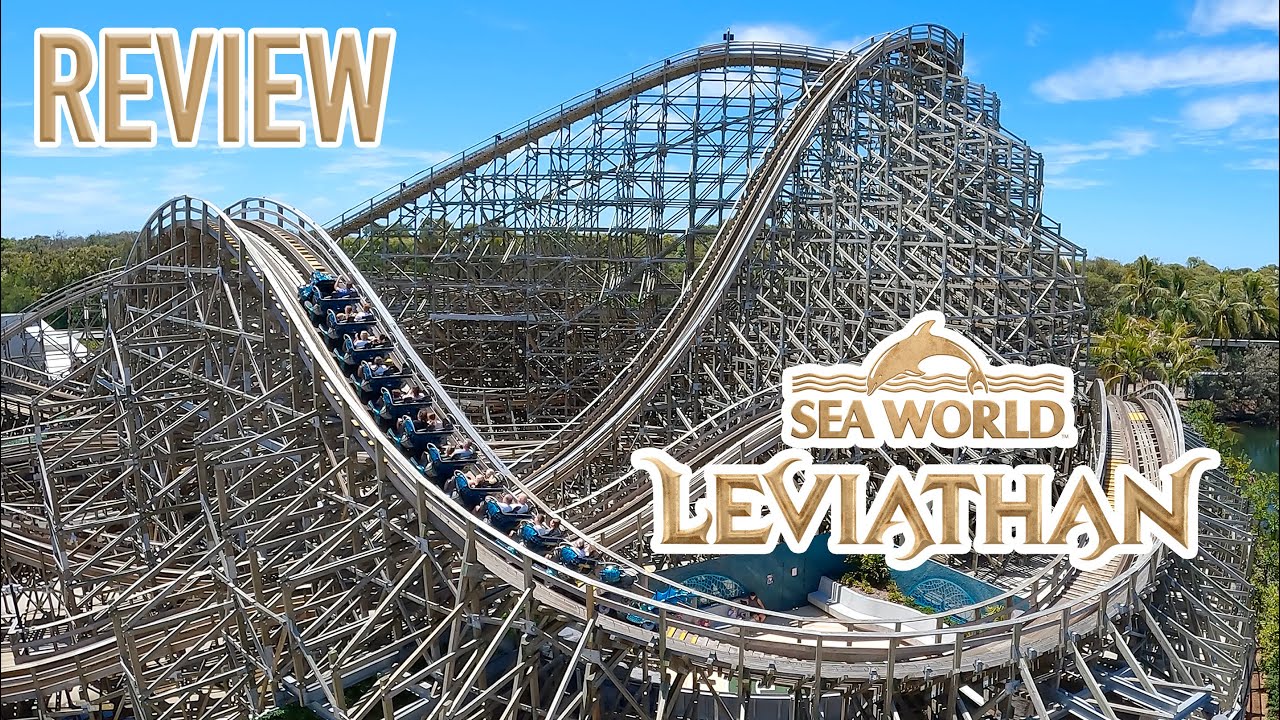This detailed photograph showcases a towering and elaborate wooden rollercoaster named Leviathan at SeaWorld. The intricate wooden framework is clearly visible, with long support beams and scaffolding holding up the high drops and curving tracks. The coaster cars, which are blue, are seen climbing a hill just left of center, poised for the next thrilling descent. The rollercoaster's track appears to be metal, embedded within the wooden structure. In the upper left corner of the image, 'Review' is written in light brown text with a white outline, while the lower right corner features 'SeaWorld Leviathan' in similar light brown text. The background displays a cluster of palm trees on the right side under a blue sky dotted with clouds, adding a touch of scenic beauty to the thrilling atmosphere.